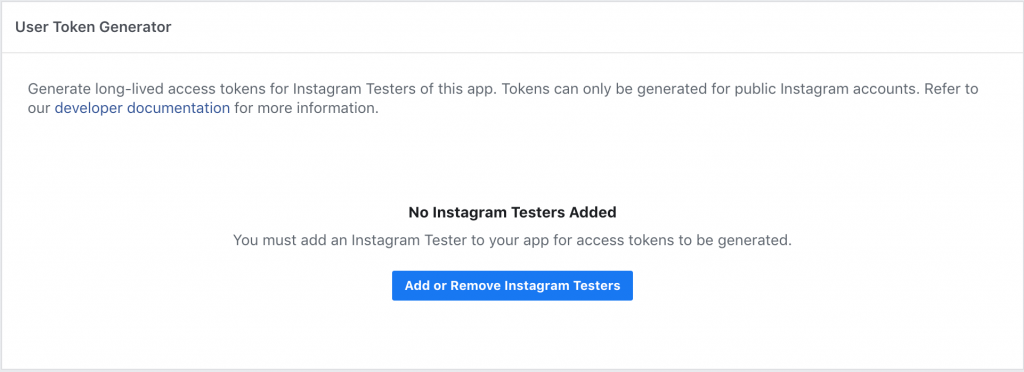The image is a landscape-oriented screenshot displaying a section of a computer screen, specifically featuring an interface element titled "User Token Generator." At the top left corner, the title "User Token Generator" is prominently displayed, with the words "User," "Token," and "Generator" capitalized. Below this title, a thin gray line stretches horizontally across the width of the image.

Underneath the line, there is a light gray text which reads: "Generate long-lived access tokens for Instagram testers of this app. Tokens can only be generated for public Instagram accounts. Refer to our developer documentation for more information." The phrase "developer documentation" is highlighted in blue, indicating that it is a clickable hyperlink.

Further down the image, centrally aligned, is a bold black text stating: "No Instagram testers added." Below this, in lighter gray text, a message reads: "You must add an Instagram tester to your app for access tokens to be generated."

At the bottom center of the image, there is a large blue oblong button containing white bold text which says: "Add or Remove Instagram Testers."

In summary, this screenshot captures a straightforward interface related to the functionality of generating user tokens for Instagram testers within a specific application. There is no additional context or background in the image.